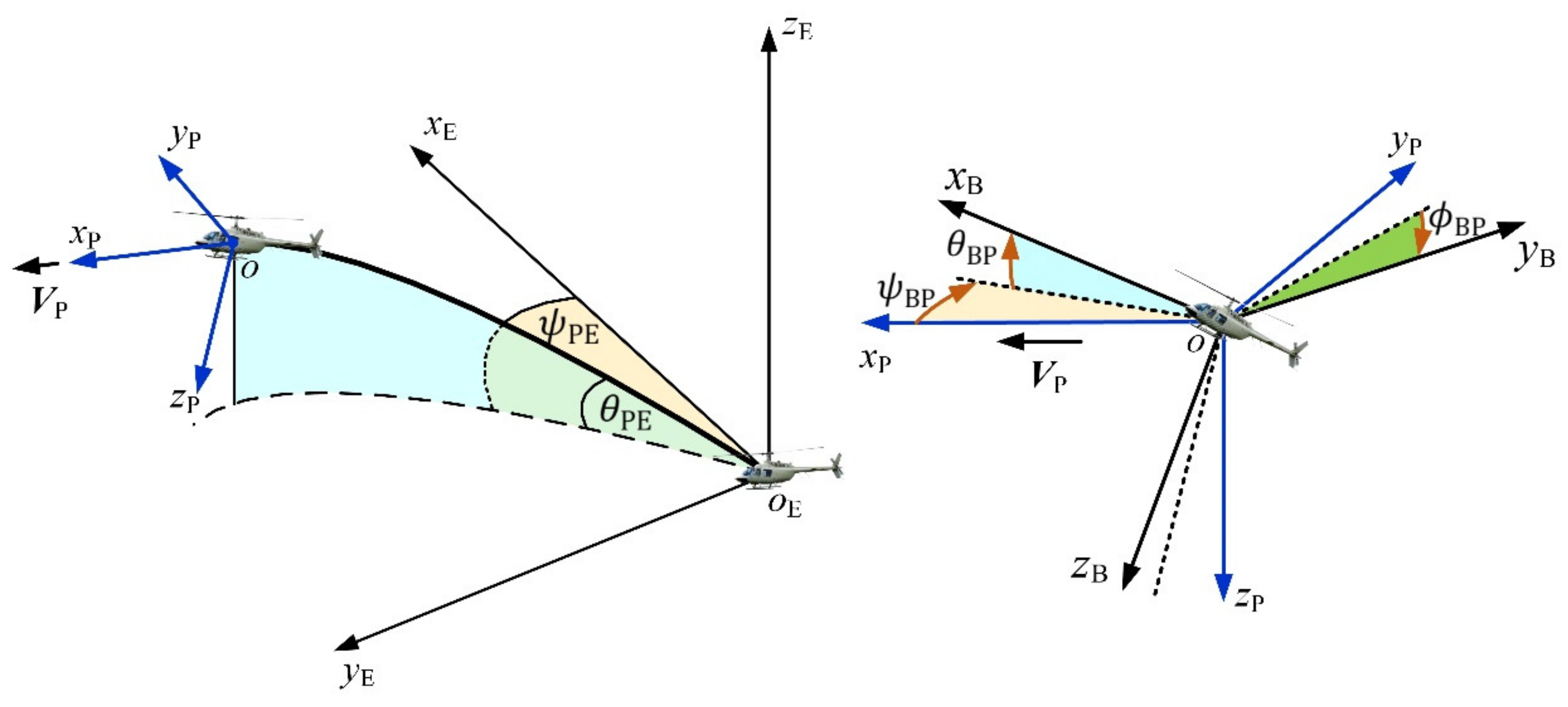The image depicts a detailed trigonometric and kinematic analysis of helicopter flight paths, illustrated with comprehensive mathematical diagrams. Central to the diagrams are three helicopters: one on the right, one on the left, and one in the center. The diagram on the left features a helicopter annotated with arcs resembling clock hands, marked with x, y, and z-axes, and demonstrates angles and potential trajectories, including paths that suggest takeoff or liftoff scenarios. Numerous colored arrows and labels, including light green, teal, and beige, alongside black dotted and solid lines, define various angles and velocity vectors. The diagram on the right presents another helicopter with several arcs labeled with Greek letters, blue and black arrows indicating angles, and detailed trigonometric angles symbolized by curved lines between solid and dotted lines. The right diagram's axes align towards 7 o’clock, 10 o’clock, and 2 o’clock, incorporating blue and black arrows and diverse color-coded annotations such as green, blue, and pink labels to emphasize various angular measurements and velocities. Additionally, a direct line connects the central helicopter to the one on the left, potentially indicating a travel path. This comprehensive portrayal underscores the intricate attack angles and trajectories calculated for the helicopters.